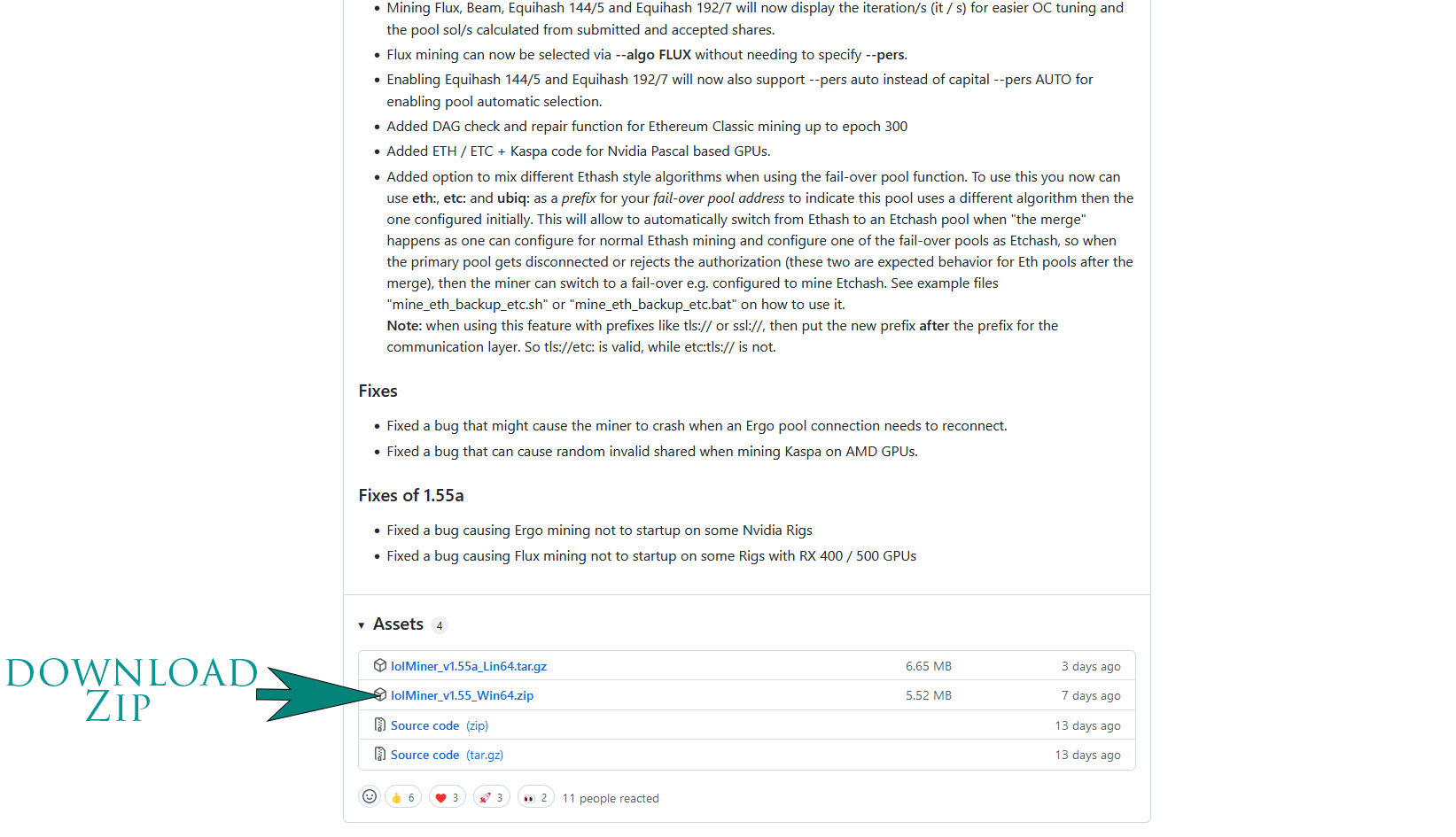A square-framed image with an all-white background showcases the detailed lower portion of a page primarily on the right side. The page contains a list of fixes for software updates, including:

- Resolving a bug that might cause the miner to crash when an Ergo pool connection needs to reconnect.
- Fixing a bug that can cause random invalid shares while mining CASPA on AMD GPUs.
- Addressing issues in version 1.55a, such as:
  - A bug causing Ergo mining not to start on some Nvidia rigs.
  - A bug preventing Flux mining from starting on rigs with RX 400/500 GPUs.

The bottom section of this outlined information page is marked with a heading "Assets," under which four blue hyperlinks offer downloadable zip files.

On the left side of the frame, a prominent green section features the text "Download zip" in green, accompanied by a large green arrow pointing towards the second asset in the list.